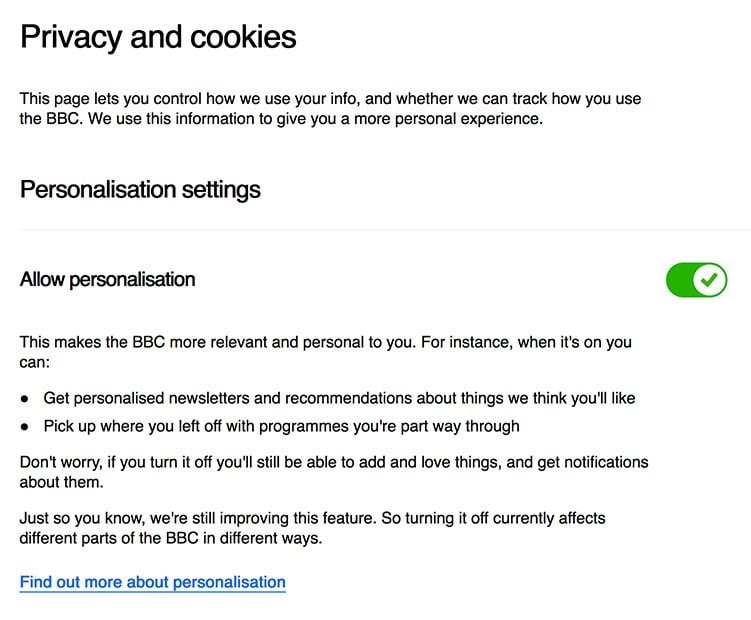**Image Description: Privacy and Personalization Control Page on BBC Website**

The image displays a white background with predominantly black text and a green slider button. 

- **Header:** In large bold text, the header reads "Privacy and Cookies."
- **Main Body Text:** Below the header, a paragraph explains the purpose of the page: "This page lets you control how we use your info and whether you can track how you use the BBC. We use this information to give you a more personal experience."
- **Subheader:** In a slightly smaller but still bold font, the subheader reads "Personalization Setting."
- **Sub-Subheader and Slider:** A smaller header labeled "Allow Personalization" appears next. Next to this is a green slider button positioned to the right. The slider has a check mark indicating that personalization is enabled.
- **Benefits List:** Two bullet points detail the benefits of allowing personalization:
  1. "Get personalized newsletters and recommendations about things we think you'll like."
  2. "Pick up where you left off with programs so you're part way through."
- **Informative Note:** Another paragraph states, "Don't worry if you turn it off; you'll still be able to add and love things and get notifications about them."
- **Closing Note:** The final paragraph notes, "Just so you know, we're still improving this feature so turning it off currently affects different parts of the BBC in different ways."
- **Interactive Link:** At the very bottom, there is blue hyperlink text that reads, "Find out more about personalization."

Overall, the image effectively communicates how users can control their privacy and personalization settings on the BBC website.